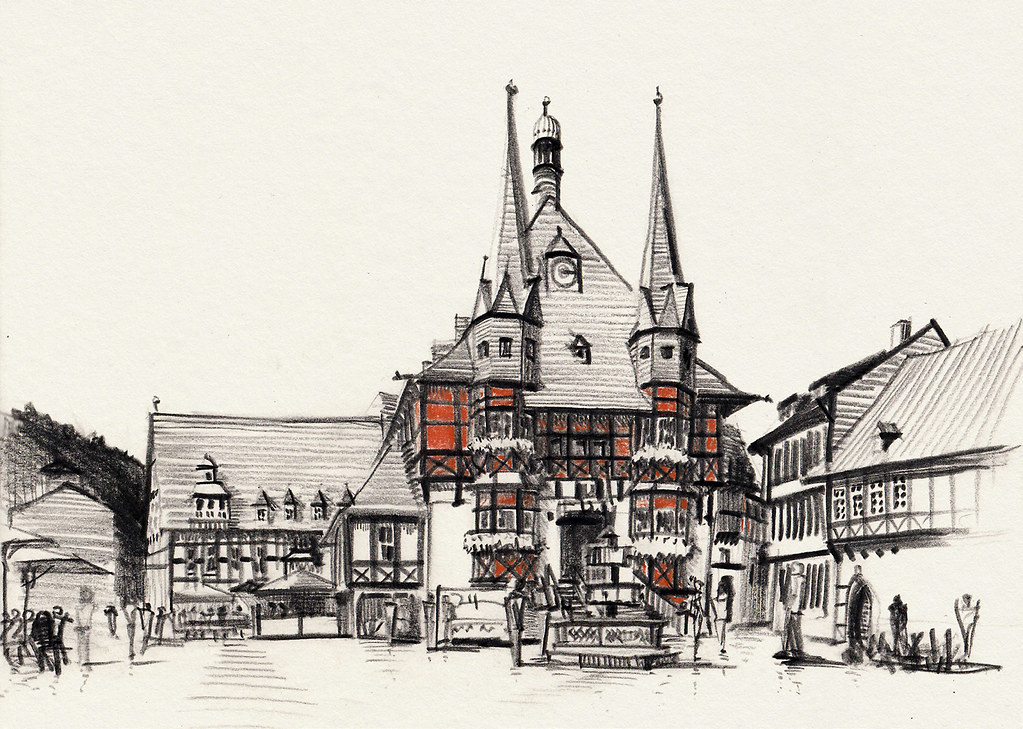This detailed drawing, executed in black pencil, depicts an old village centered around a grand castle. The castle stands out with its two steep spires, a pointed dome at the top, and a large front stairway. Its numerous front-facing windows are uniquely colored in a striking burnt orange. The castle roof features a clock and is topped with what appears to be a watchtower. Surrounding the castle, there are smaller buildings and various people walking around, suggesting shops and restaurants. Specific left-side details include a pavilion and a picnic table with an umbrella, indicating a communal area. Flowers adorn the scene, and an arched door is visible in one of the side buildings, enhancing the quaint village atmosphere. The entire sketch is rendered in a monochromatic palette, with the exception of the vividly colored windows, and the sky above is depicted in shades of gray.